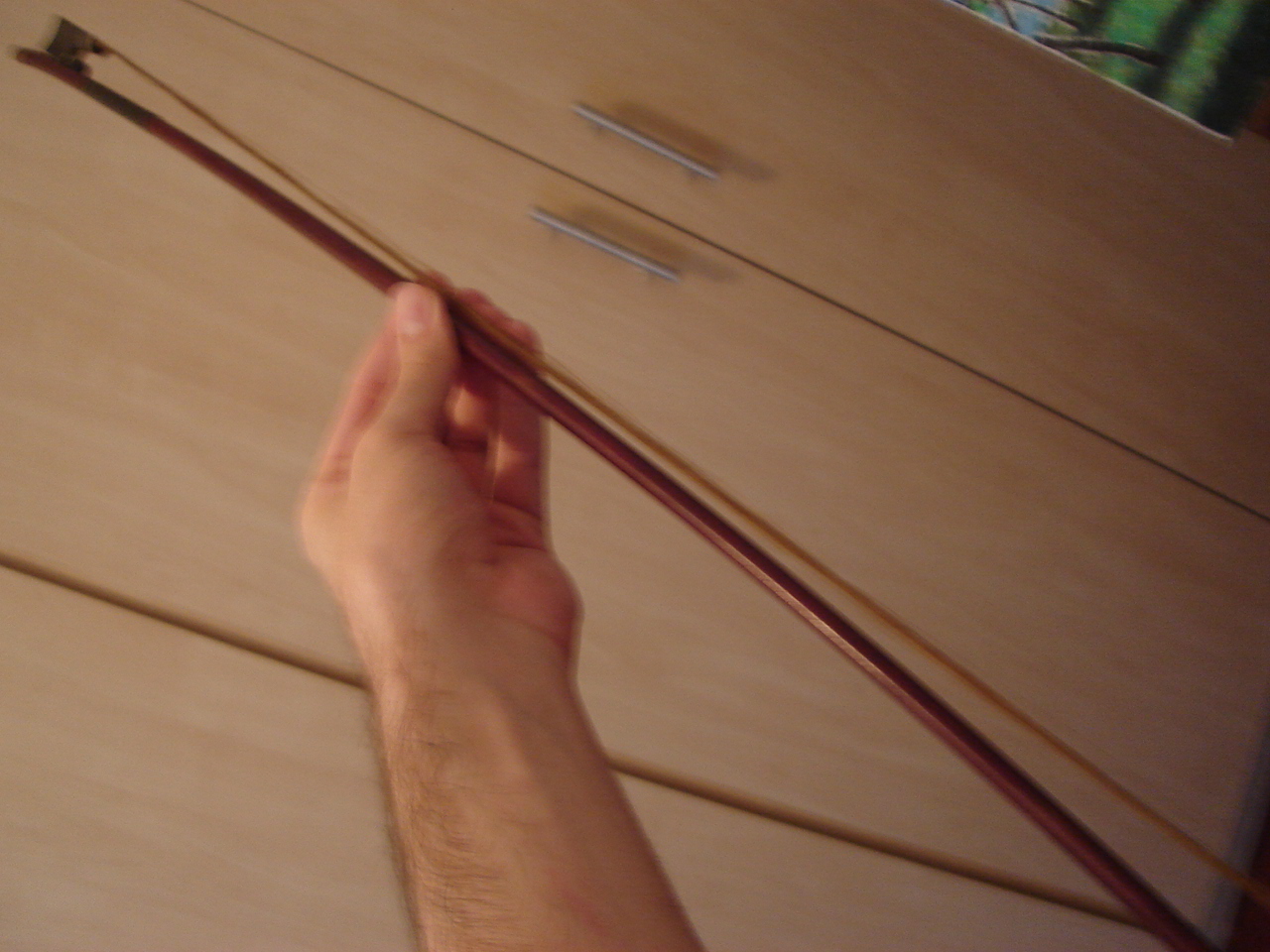The image depicts a grainy, out-of-focus close-up of a man's left hand, prominently featuring very white skin and a notably hairy arm. The hand, seen from just past the wrist upwards, holds a violin bow, characterized by a reddish-brown wood color. The bow is clasped between the thumb on one side and the four fingers on the other. The photograph is captured at a diagonal angle. In the blurred background, a light wood dresser with silver drawer pulls is visible. The pulls are positioned closely together, with one at the bottom of the top drawer and the other at the top of the lower drawer. Additionally, a part of a green curtain appears in the top right corner of the image.